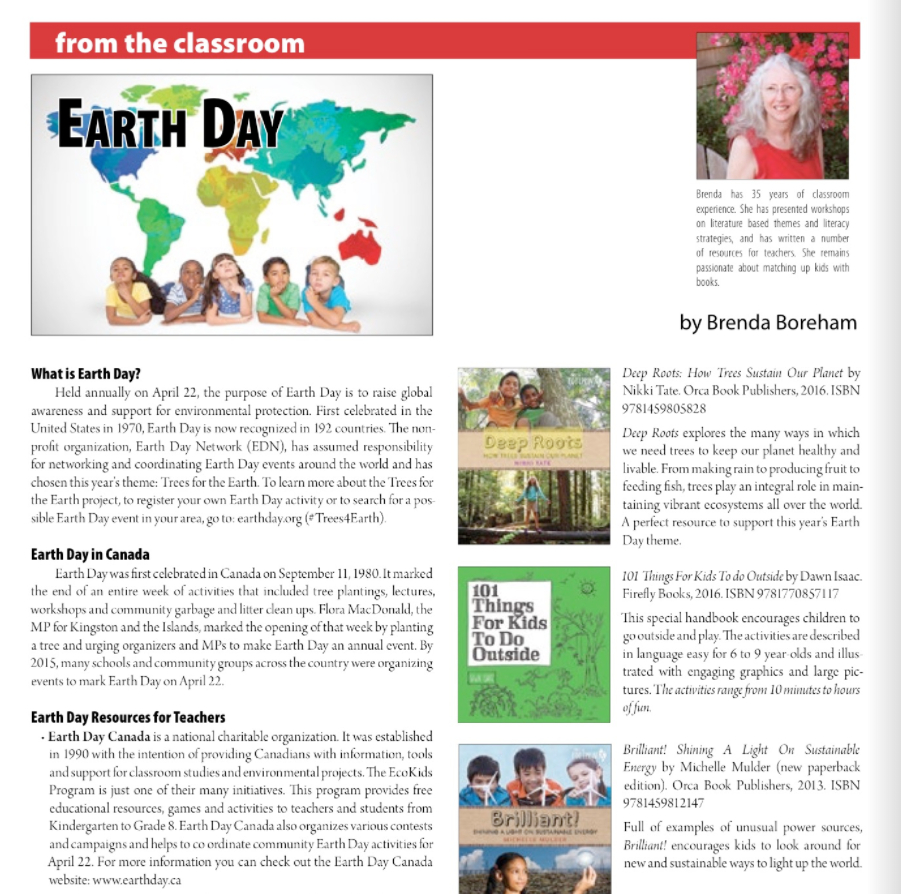In this image, we see what appears to be a page from a book or magazine. At the top, there is a red bar with the phrase "from the classroom" written in all lowercase letters. The rest of the page has a white background suggesting its origin from print media.

On the top left, right underneath the "from the classroom" heading, there is a picture of five children sitting in a row. Each child has one arm under their chin and the other arm resting on their lap. The children, arranged from left to right, are a girl, a boy, another girl, and two boys. Above them, in large, bold, capital letters, it reads "EARTH DAY." Behind the children is an illustrated depiction of the Earth, with visible continents color-coded: North America in blue, South America in green, Africa in lime green, Europe in orange, Asia in greenish-blue, and Australia in red. Notably, Antarctica is not visible in this depiction.

To the far right of the children's image, there is a photograph of an older Caucasian woman, likely in her 60s. She has long, curly, predominantly white hair, and is wearing glasses. She is sitting behind a bed of pink flowers, and is dressed in what appears to be a red tank top or dress. The woman has a warm smile on her face. A small caption identifies her as "Brenda," noting she has "35 years of classroom experience." The text also attributes the article to Brenda Boerheim, indicating she is the author.

The page also includes several paragraphs with headers: "Earth Day," "Earth Day in Canada," and "Earth Day Resources for Teachers." Each section provides descriptions related to these topics.

On the right, there is a column dedicated to reference books, listing and displaying images of three titles: "Deep Roots," "101 Things for Kids to Do Outside," and "Brilliant." These books are recommended as resources for further reading.